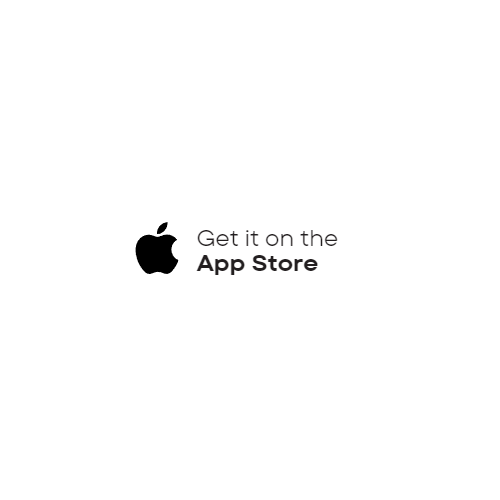The image features a minimalistic and clean design with a white background that seamlessly blends into the surrounding page. Central to the design is a black Apple icon, distinguished by its leaf pointing towards the top right and a recognizable bite taken out of its right side, symbolizing the tech company Apple. To the right of the iconic Apple logo, the phrase "Get it on the" appears in regular black font. Directly below this, in a more bolded black font, is the text "App Store." The entire image uses only black and white, with no other colors, additional pictures, or text. The simplicity and clarity of the design emphasize its minimalistic appeal.